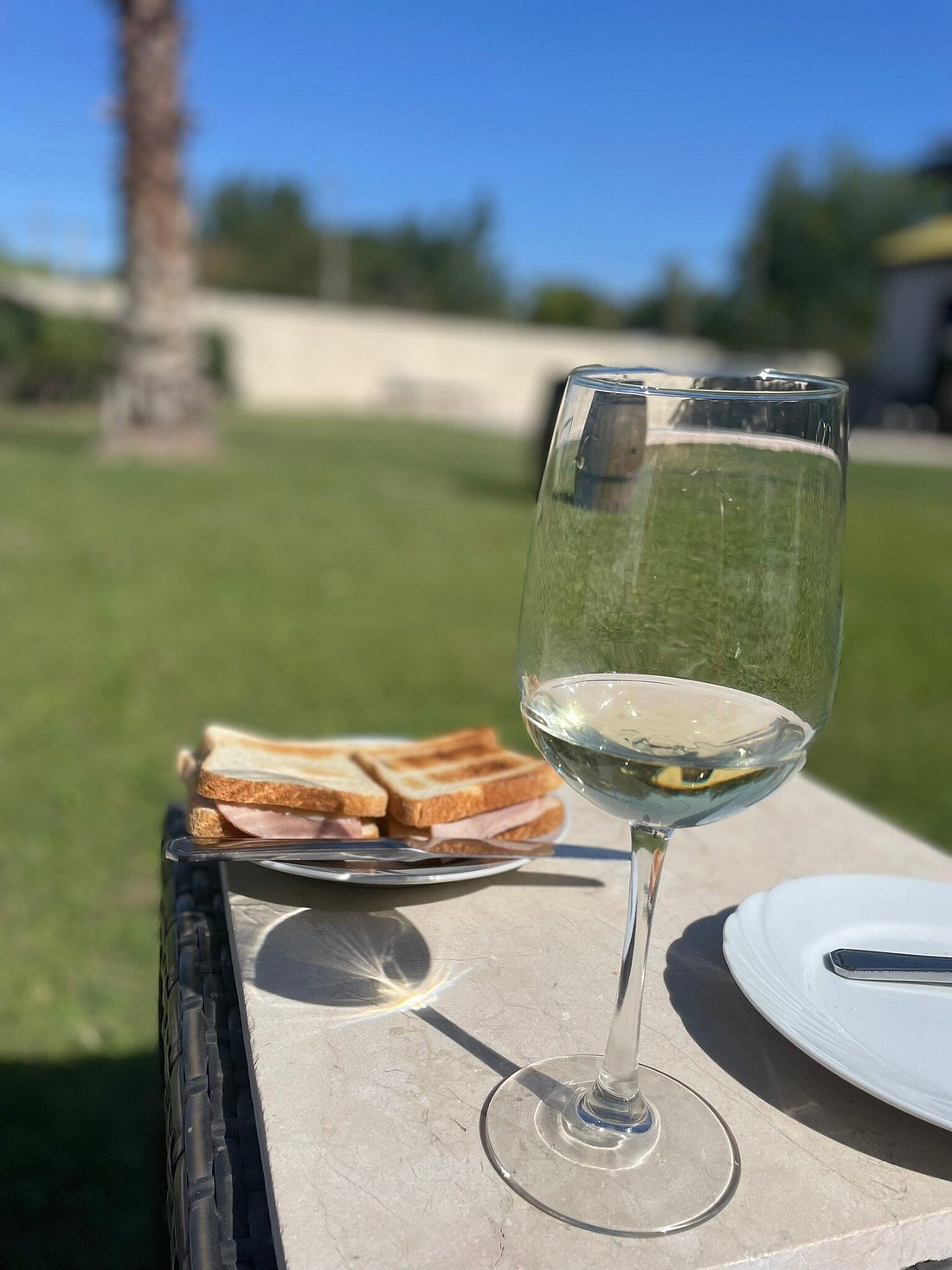In the foreground of the image, a glass of clear water—likely in a wine glass—sits on an outdoor stone table with a white top, accented by the shadows of neighboring objects. The table rests on a large green lawn, bordered on one side by a white fence, with green bushes growing in front. A tall, partially visible brown tree trunk extends upwards, its top cut off from the frame. The background is blurry, showcasing a mix of blue sky and green trees, suggesting an early afternoon setting. 

On the table, two white plates are visible. One plate holds two toasted ham sandwiches, with a silver butter knife resting atop, while the other plate appears empty but for a piece of silverware partially cut out of the image. To the right of the frame, there’s a hint of a housing area featuring a yellow roof and white siding. The overall ambiance appears to be that of an outdoor picnic lunch, peaceful and relaxed.